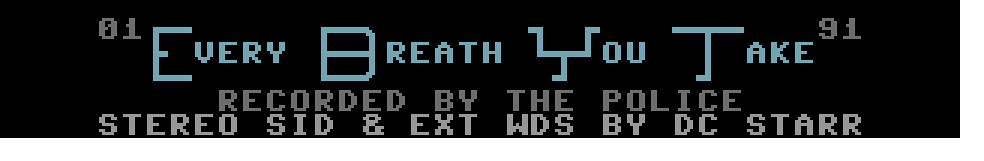This image features a long rectangular banner with a black background. Dominating the banner is the song title "Every Breath You Take" in light blue text, with the first letters, E, B, Y, and T prominently capitalized. Flanking the song title, "01" appears in gray on the top left, and "91" on the top right. Right below the main title, in a dark gray color, it states "Recorded by the Police." Beneath this, in a slightly lighter gray text, it reads "Stereo SID and EXT WDS by DC Starr," noting that "Starr" has an extra "r." This detailed information suggests it's identifying the song along with additional production or remix credits.